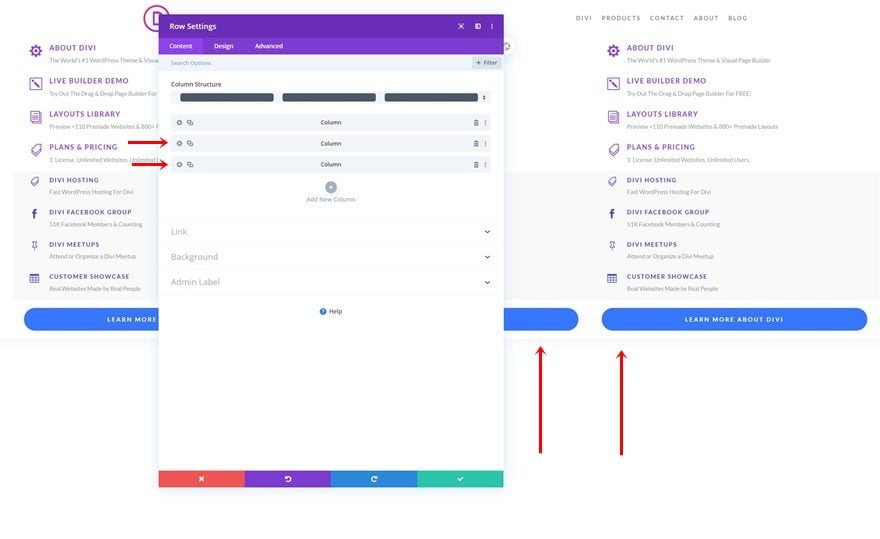The image depicts a page organized into two distinct columns. The left column contains sections labeled "Plans" and "Pricing," with additional details in a lighter font below them. The right column contains another row with eight pieces of information. Superimposed on this page is a prominent rectangle with a purple border at the top, labeled "Settings" or "Row Settings." This rectangle features three icons beneath the label and a lighter purple border containing three pieces of information in white text. Below this border are six different sections, each with three black bars displaying "0%" on them. Additionally, there are two red arrows pointing from the elements in the left column towards the second bar of information within the superimposed rectangle.